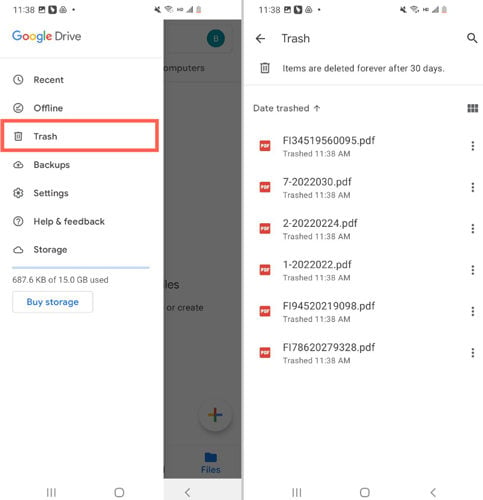The image appears to be a side-by-side screenshot of two different phone screens displaying sections of the Google Drive app. 

**Left Screen**: The upper portion of the screen displays the Google Drive home interface. At the top, the title "Google Drive" is visible, along with a list of menu options: Recent, Offline, Trash, Backup, Settings, Help and Feedback, Storage, and a blue "Buy Storage" button at the bottom. Each option is listed in a vertical format, with the "Trash" option highlighted by a red outline, indicating it is currently selected.

**Right Screen**: This screen showcases the contents of the "Trash" section in Google Drive. At the top, "Trash" is labeled beside a back arrow and a search icon. Below that, a message states, "Items are deleted forever after 30 days," serving as a reminder of the permanent nature of this section. There is also a "Date Trashed" header that organizes the deleted items. The screen displays six PDF files marked as trashed, each accompanied by a vertical three-dot menu icon on the right, giving additional functionality such as restoring or permanently deleting the items.

Both screens share common elements at the top including the clock showing "11:38," Wi-Fi signal strength, sound being muted, and the battery icon indicating the phone's charge status.

This detailed comparison highlights the Google Drive's navigation interface and the specific functionalities of the "Trash" section, offering an insightful glimpse into the app's user experience.